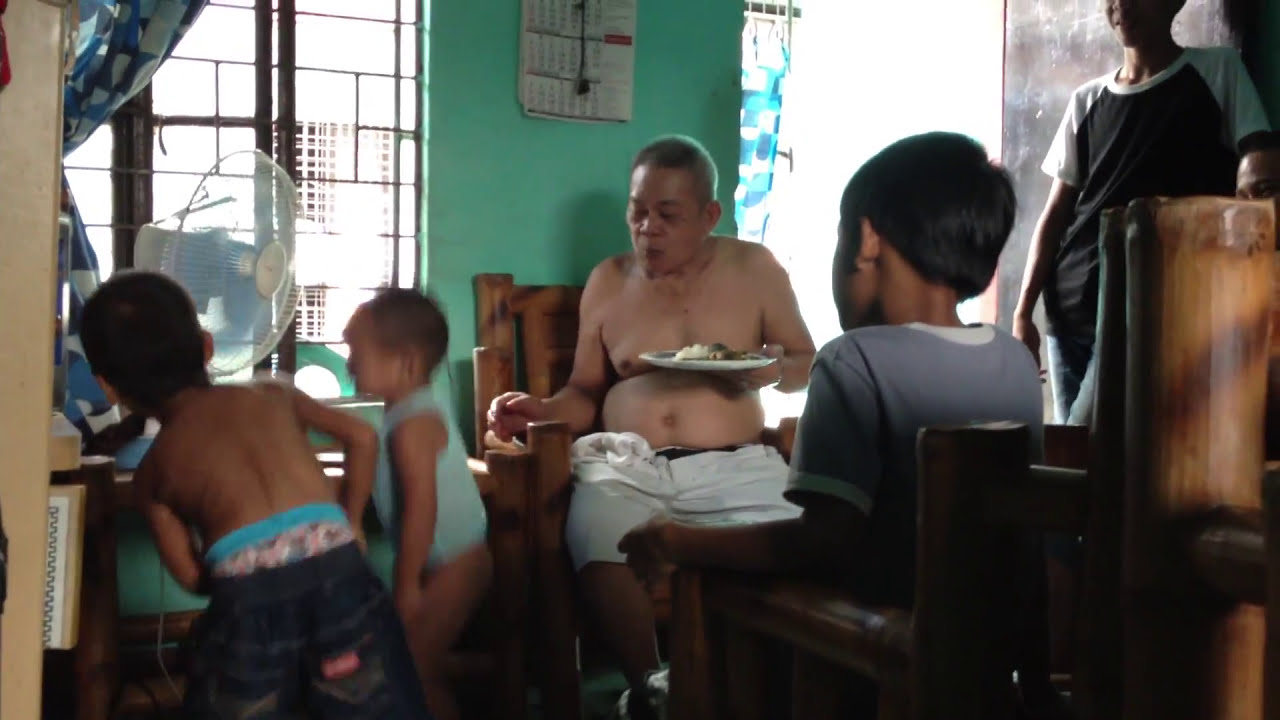In this image, there's an Asian family gathered in a modest room with noticeable green walls adorned with a paper calendar. The central figure is an older gentleman, possibly in his 50s or 60s, with gray hair and a pot belly, sitting shirtless in a wooden chair while eating from a white plate. Surrounding him are multiple people, including three young boys: one around 9 or 10 years old standing near the fan, another about 5 or 6 years old wearing a green tank top and underwear, and the youngest, about 4 years old, wearing blue jean shorts and no shirt. A teenage boy, thin and dressed in an old-fashioned outfit, stands nearby. Additionally, there's another adult standing to the right of the older man, and another person partially visible, sitting off to the right-hand side. The room features blue curtains on the windows, a plug-in stand-up fan, and a few wooden chairs scattered around. Light filters in from an open doorway, adding to the cozy but slightly cluttered ambiance of the space.